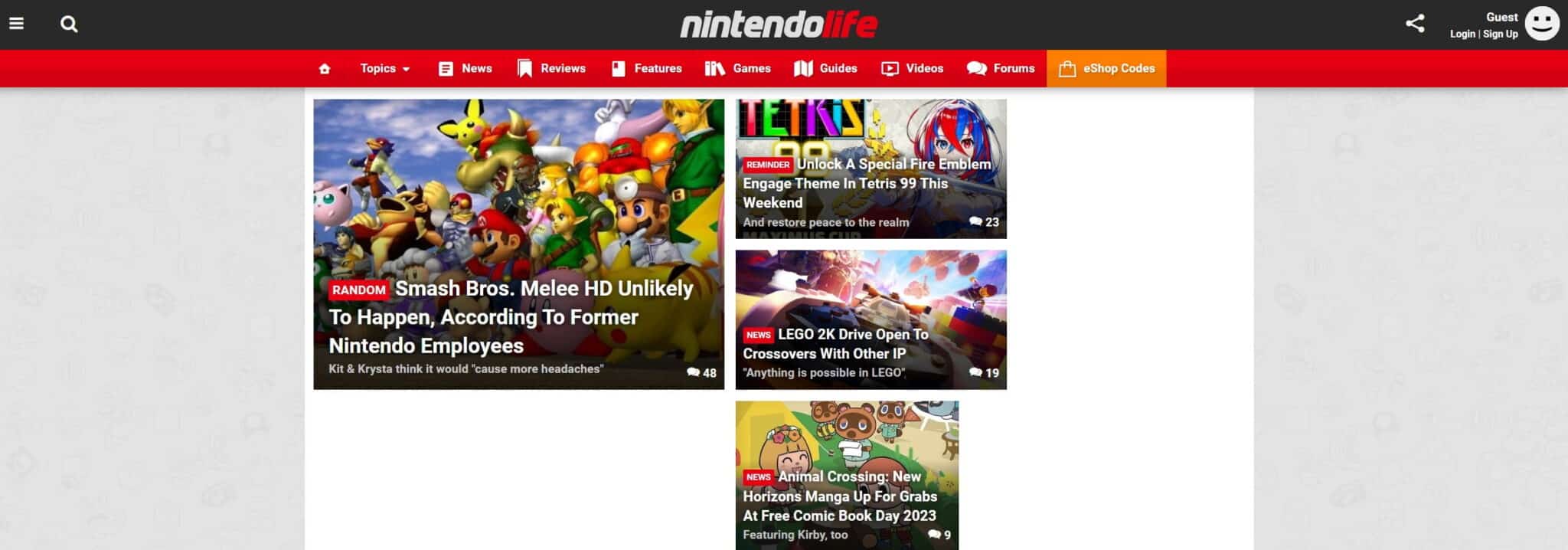Here we have a screenshot of the Nintendo Life website. The layout starts with a dark gray banner along the top, featuring a magnifying glass icon on the left, indicating a search function. Centrally positioned in the banner is the site’s name, "Nintendo Life,” while the right side displays a smiley face icon next to the labels "Guest" and "Login / Sign Up."

Directly below this, a red navigation bar extends from the center-left to the center-right, providing several options: Home, Topics, News, Reviews, Features, Games, Guides, Videos, Forums, and an orange icon of a briefcase labeled "eShop Codes."

The main content area is divided into sections. Flanking this section are two thin, gray rectangular banners on the far left and right sides. The central portion of the page is white and showcases featured articles. 

On the far left, there is a larger featured article box displaying a montage of famous characters from the Mario franchise. The headline reads, "Random: Smash Bros. Melee HD Unlikely to Happen According to Former Nintendo Employees," with a subtext explaining, "Kit and Krista think it would cause more headaches." This article has garnered 48 comments.

To the right of this large article are three smaller articles stacked vertically:
1. "Unlock a Special Fire Emblem Engage Theme in Tetris 99 This Weekend and Restore Peace to the Realm," with 23 comments.
2. An article about Lego, which has 19 comments.
3. A piece discussing Animal Crossing, which has received 9 comments.

This detailed structure provides a clear and informative snapshot of the Nintendo Life website’s homepage layout, capturing the key features and current highlighted stories.